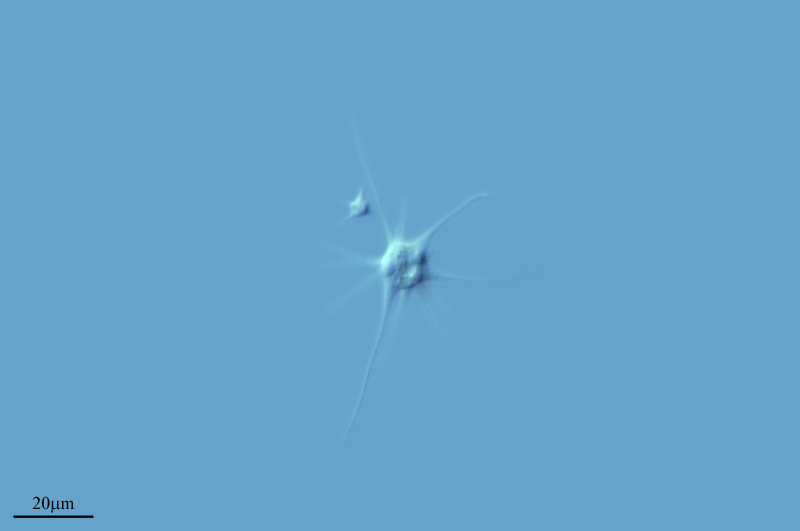The photograph features an artwork dominated by a large, bright powder blue square. In the center of this solid blue expanse, there is a raised, protruding section that appears as if material was pushed from behind, creating a wrinkle or dent-like effect. This raised area is the same shade of blue as the rest of the square, though it includes lighter blue and white streaks, reminiscent of cellular growth observed under a microscope, with tendril-like extensions radiating from the main protrusion. To the left of this central raised spot, there's a smaller, similarly designed area with additional tendrils. The only textual element in the image is located in the lower left corner, displaying the black characters "20 U.M." There is otherwise no identifying information or other objects present in the photograph.